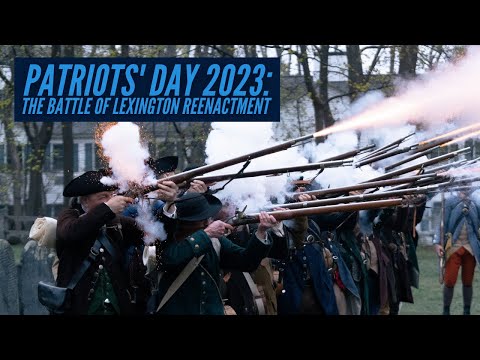The image is a low-resolution still frame that appears to be a thumbnail for a YouTube video, presented in a landscape layout with black bars at the top and bottom. It showcases a line of at least 20 men, dressed in blue Revolutionary War-era uniforms complete with tricorn hats, long coats with multiple buttons, and holding flintlock-style muskets. All of the men are firing their muskets into the air, creating a thick plume of smoke behind them. Off to the side, there is one individual also in a blue uniform, casually resting a rifle on his shoulder. In the upper left-hand corner, a dark blue rectangle features light blue text that reads, “Patriot's Day 2023, the Battle of Lexington Reenactment.” The backdrop includes historical or residential buildings, characterized by a large white structure with numerous windows and blue accents, set against a line of trees. This scene vividly captures the atmosphere of a Revolutionary War reenactment.